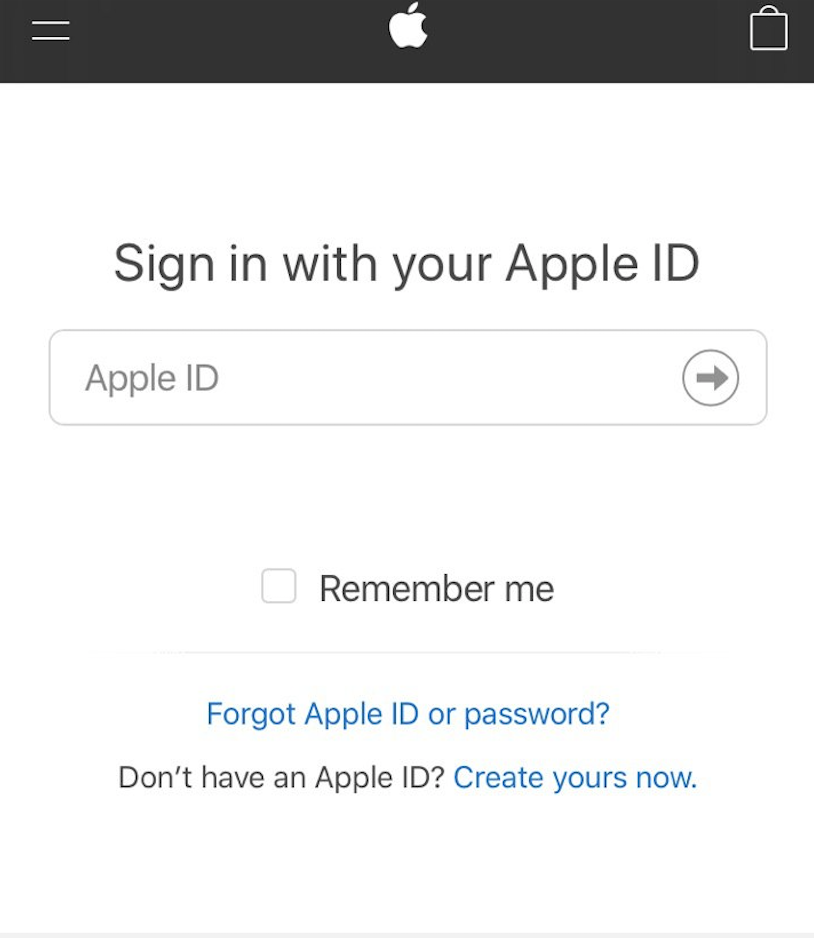The image appears to be a screenshot taken from a cell phone, displaying a zoomed-in view of an Apple ID sign-in page. 

At the top of the screen, a black rectangle is visible, featuring a white Apple logo with a bite taken out of it. To the right of the logo, there is a white icon resembling a bag with a handle, also associated with Apple.

Below these icons, the screen shows a large white space with black text that reads, "Sign in with your Apple ID." Beneath this text is a rectangular input field labeled "Apple ID," where users can enter their credentials. 

To the right of this input field, there is a small circle containing a gray arrow pointing to the right, suggesting the action of proceeding or submitting the entered Apple ID.

Further down the page, there is another white space containing a gray checkbox with black text next to it that says, "Remember me." 

A faint gray line separates this section from the next.

In the lower part of the image, there is a blue link reading "Forgot Apple ID or password?" followed by another line of text in black that asks, "Don't have an Apple ID?" with a subsequent blue link stating, "Create yours now."

The bottom of the image is marked by another faint gray line, completing the structured and user-friendly design of the Apple ID sign-in page.